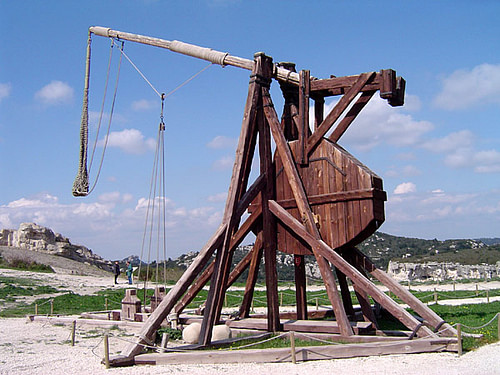This outdoor photograph captures a distinct and somewhat surreal landscape dominated by a substantial wooden trebuchet, standing approximately 25 feet tall. The trebuchet, constructed from brown wood, has tall legs and sturdy support beams with a circular structure in the middle, from which several pillars and ropes extend. A light wood-colored arm extends back and to the left, with something attached to its end. The device is situated on a patchy terrain consisting of light-colored sand, gray rocks, and lush green grass.

The scene is set under a clear blue sky, adorned with gray and wispy white clouds. In the backdrop, distant mountains and verdant green trees enhance the natural beauty of the landscape. Far off in the distance, two individuals can be seen conversing; the person on the left is dressed in black, while the one on the right wears blue. The photograph interestingly combines elements typically seen at a beach with features of a dry, grassy environment, making it a unique and captivating image.